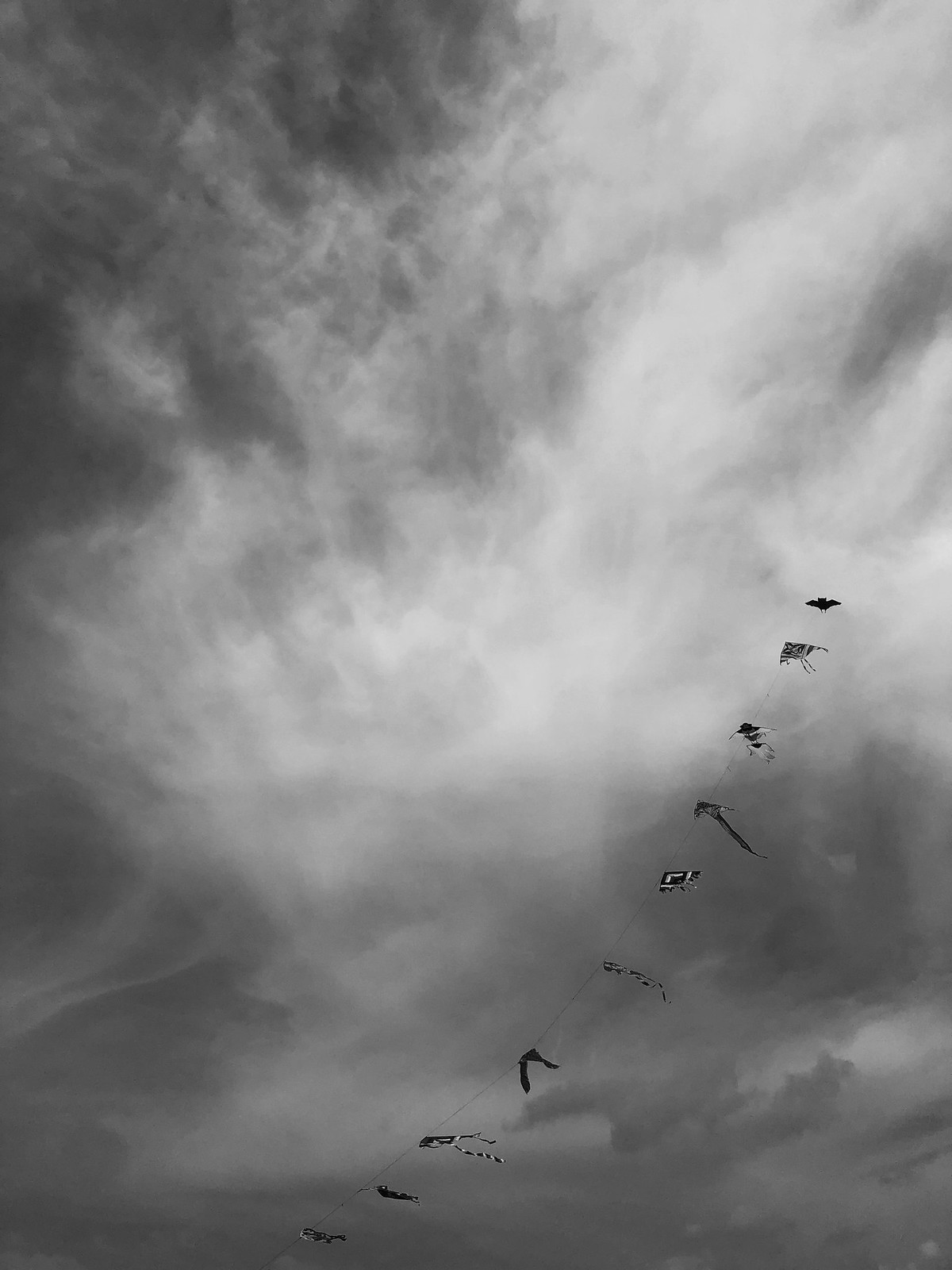The black-and-white image, possibly a photograph or a detailed drawing, captures an ominous night sky filled with a gradient of dark and lighter clouds. Stretching diagonally from the bottom left corner to the upper right middle, a single string is adorned with approximately 10 individual kites. These kites, spaced apart every five feet or so, exhibit a variety of shapes and designs. Some are long and slender, while others are more triangular, with some resembling creatures like butterflies, moths, and even a frog. The final kite at the top prominently appears as a black bat, adding a distinct, eerie touch to the composition. The use of monochrome enhances the overall dramatic and surreal atmosphere of the scene.